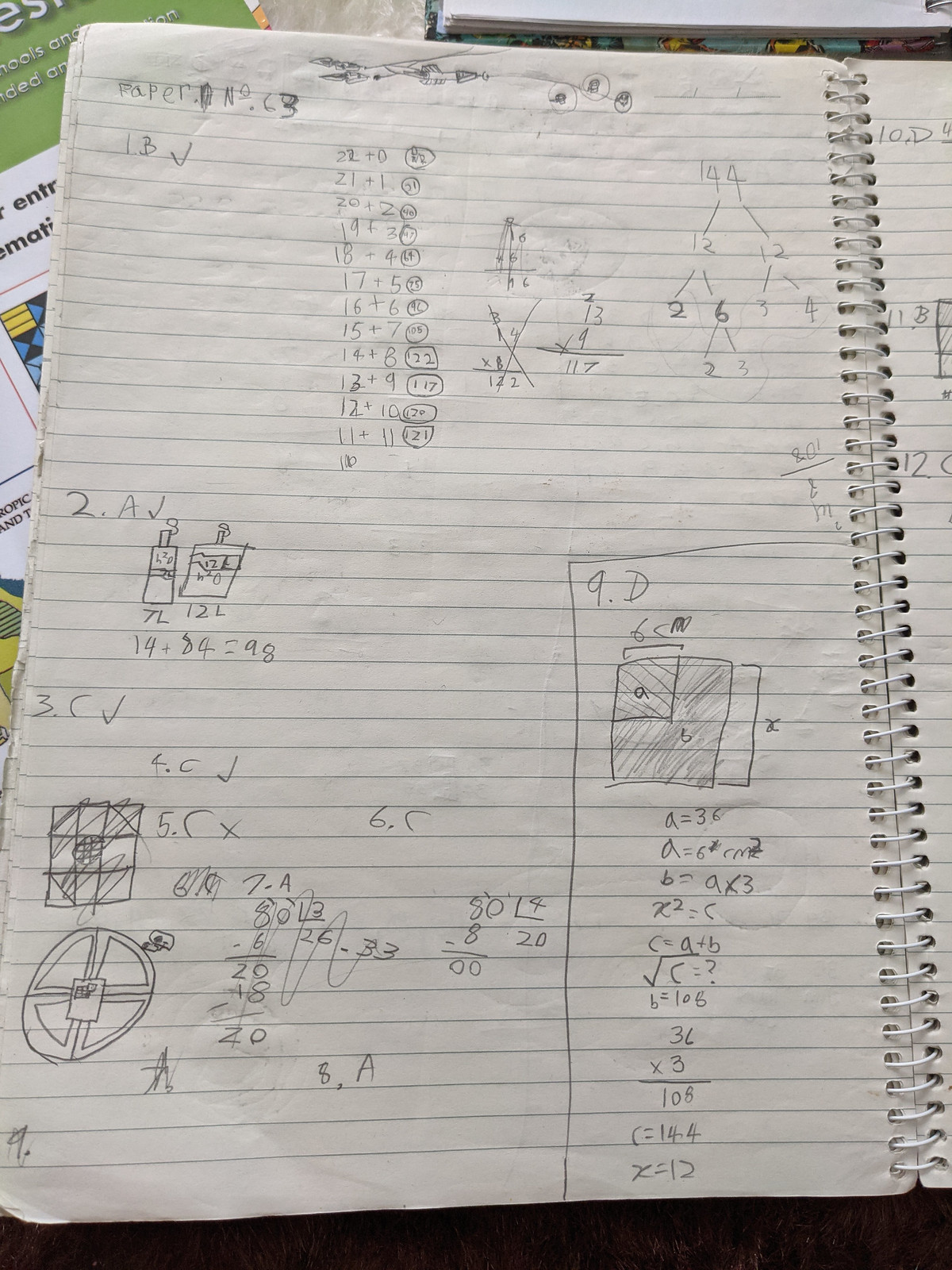A detailed caption for the image might be:

"An open spiral notebook, commonly used in schools, is displayed with its left page prominently visible. This page is a standard piece of lined school paper, filled with the meticulous handwritten notes and calculations of a math student. At the top center of the page, a long line of numbers is shown being added together, indicating a step-by-step approach to solving math problems. Scattered across the page are various mathematical problems, including addition, subtraction, potential algebraic expressions, and fractions, highlighting the diverse range of topics the student is working through. This detailed snapshot showcases the student's organized method of tackling their math homework or studying for an upcoming test, using the paper as a workspace to guide their thought process and calculations."